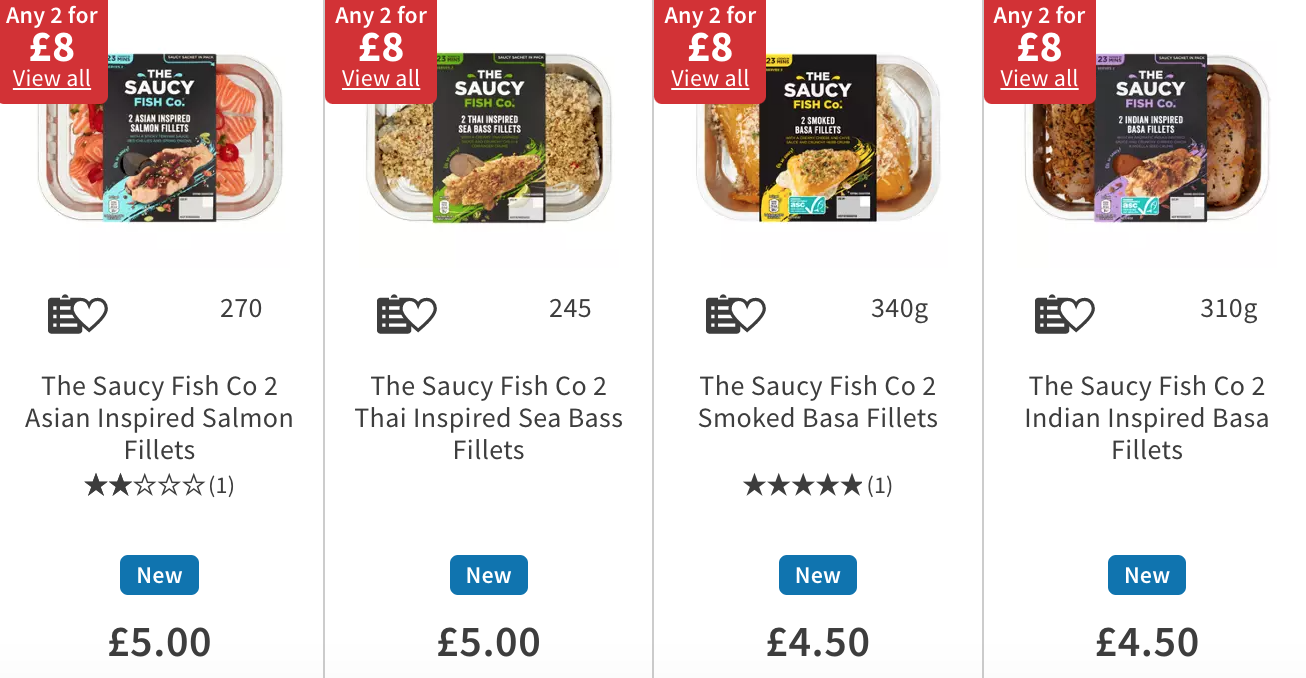Caption: 

In the grocery store aisle, a variety of seafood products from "The Saucy Fish Co." are displayed in a clean, organized row. Four different items are presented, each in a rectangular package with a line dividing them. 

1. **Asian Inspired Salmon Fillets**: The package features the label "The Saucy Fish Co." and indicates it is Asian-inspired. It highlights a special offer with a red box on the upper left corner stating "Any two for £8". The product costs £5 and has received two stars based on one review. A blue "New" label is prominently placed on the package.
   
2. **Thai Inspired Sea Bass Fillets**: Another offering from "The Saucy Fish Co.", this package looks similar and also advertises the "Any two for £8" deal. Priced at £5, it sports a blue "New" label, just like the previous item.
   
3. **Smoked Basa Fillets**: This package deviates slightly by having garnered a better rating, boasting five stars from one review. It is priced at £4.50 and also features the familiar "Any two for £8" promotion in the red box.

4. **Indian Inspired Basa Fillets**: The final product on display, identified as Indian-inspired, follows suit with an "Any two for £8" deal. It costs £4.50 and comes without any reviews or ratings displayed on the packaging.